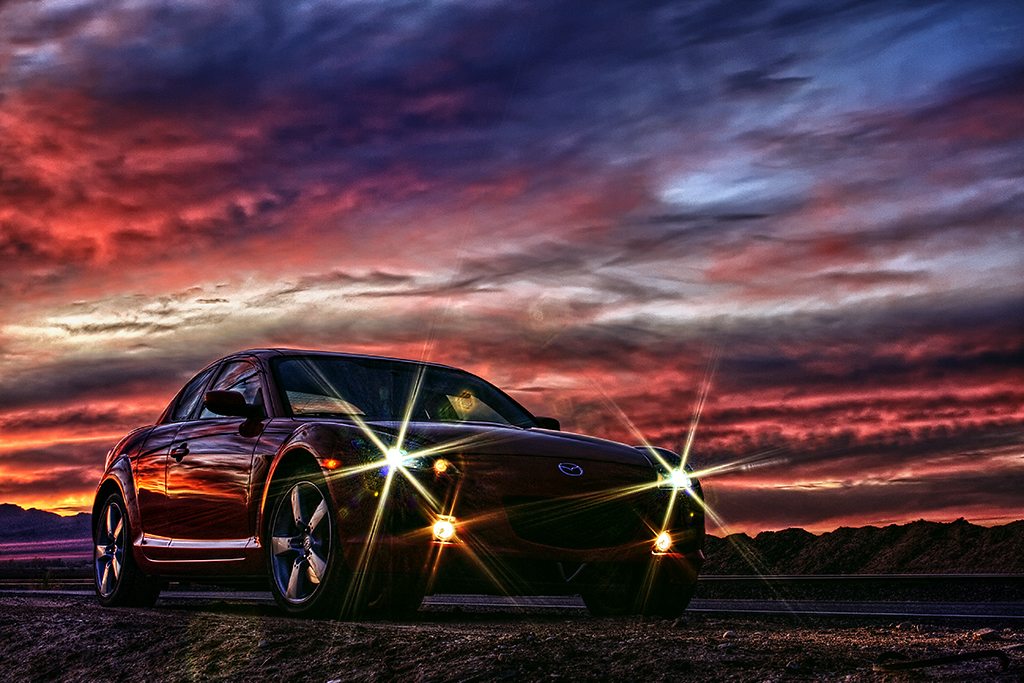This highly edited, color photograph taken outdoors at sunset captures a striking scene in landscape orientation. Dominating the lower left corner is a sleek, shiny, dark red Mazda coupe with its headlights and fog lights on, emitting dramatic starburst effects. The car, which features a silver Mazda emblem on its hood, is parked on a small gravel path beside a dark asphalt road. Occupying most of the image, the sky is a vibrant canvas of stormy clouds colored in brilliant strands of dark gray, red, orange, and cream, accentuating the dramatic atmosphere. Beneath this opulent sky, a low-lying ridge with silhouetted trees lines the horizon, providing a natural frame to the car and the richly edited sunset. The photograph's representational realism is enhanced by special filters, creating an almost surreal depiction of the scene.